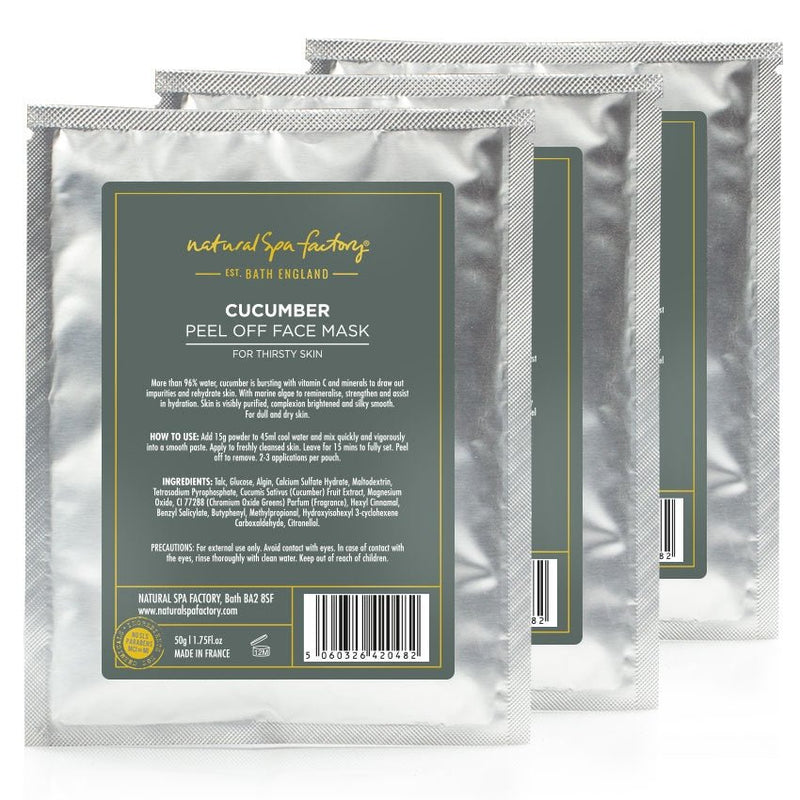The image is a product advertisement featuring three silver, square Mylar packages of the "Natural Spa Factory Cucumber Peel-Off Face Mask for Thirsty Skin." The packages are arranged with slight overlap against a plain white background, emphasizing their shiny, reflective surfaces. Each package displays a large rectangular vertical sticker in a green-gray color with a thin yellow border, prominently featuring the brand name "Natural Spa Factory" in cursive at the top, accompanied by "Established Bath, England" beneath it. Central to the label, in white lettering, is the product name: "Cucumber Peel-Off Face Mask for Thirsty Skin." The sticker also includes three paragraphs detailing the ingredients, instructions for use, and product information, along with a caution notice. Additional details such as a large rectangular barcode, a URL for the company website, the statement "Made in France," and a gold emblem in the lower left corner are also present on the label, contributing to the comprehensive and informative packaging design.